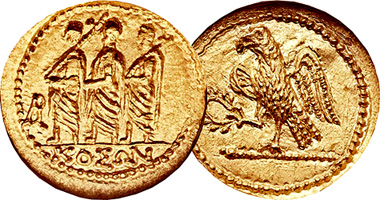The image depicts two ancient coins set against a white background, allowing for clear focus on the coins themselves. Both coins are made of a dark golden material, possibly gold or bronze. The coin on the left features three robed figures facing to the left, appearing to carry objects possibly resembling rifles over their shoulders. Underneath these figures is an inscription, "K-O-Z-A-N." The details on this coin are deeply imprinted, suggesting significant age and craftsmanship. The coin on the right showcases an eagle perched on a branch or pole, with its wings partially spread and holding laurels in its claws. Both coins are adorned with circular patterns that frame the detailed imprints, enhancing their ancient and intricate appearance. The overall presentation emphasizes the coins as historical artifacts with embossed designs rather than mere surface images.